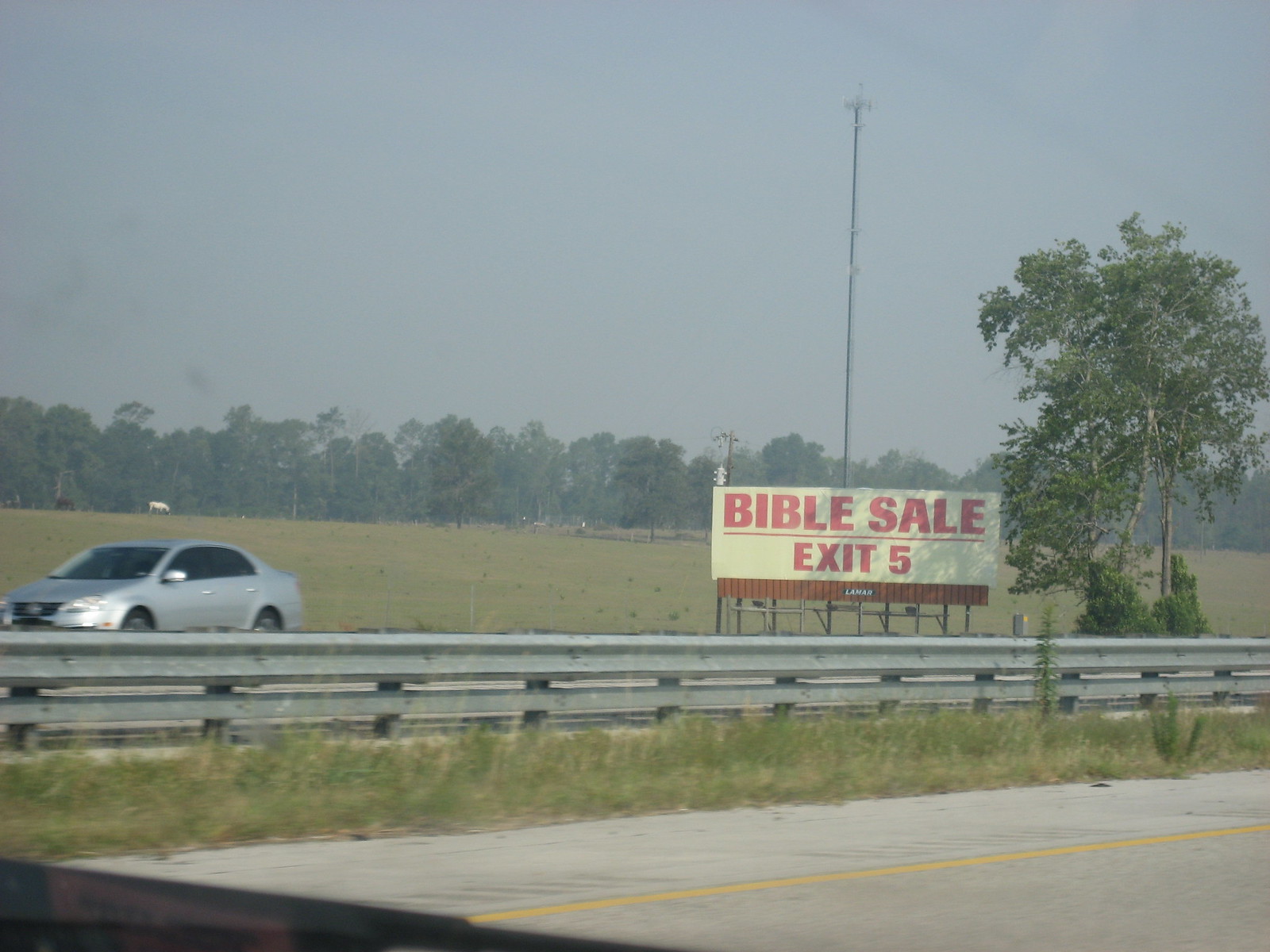The image captures a highway scene, viewed from inside a moving car, evident by the visible yellow lines on the road. A prominent billboard with a white background dominates the roadside landscape. The billboard bears the text "BIBLE SALE" in bold red capital letters, underlined with a red line, followed by the direction "Exit 5" beneath it. 

In the foreground, a sturdy guard rail extends parallel to the road, featuring a large top bar and a smaller one underneath. Beyond the rail, the grassy landscape is untamed, with tall weeds and possibly wheat stretching across the field. The scene recedes into a backdrop of deciduous trees, forming a dense line that marks the horizon.

On the extreme left edge of the image, a silver Honda, possibly in motion, suggests the ongoing traffic on the highway. A telephone pole rises directly behind the billboard, juxtaposed with a cluster of vertical trees and several bushes to its right. The juxtaposition of nature and signage paints a vivid picture of this rural highway stretch.